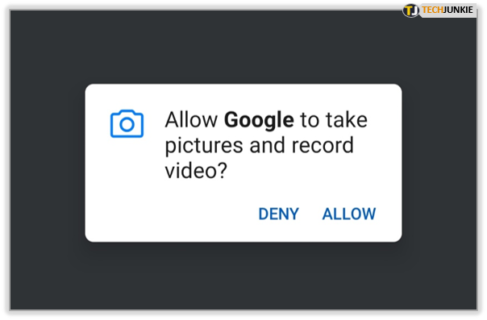The image depicts a primarily black background with a central black square faintly outlined in gray on the top, each side, and the bottom edges. Surrounding the square, the background is white on all sides. In the top right corner of the black square, there is a gray banner with the text "TECH" written in capital yellow letters and immediately adjacent, "JUNKY" in capital black letters, forming the word "TECHJUNKY." To the left of this banner is a circle, outlined in gray and filled in black, featuring a yellow "T" and a white "J" representing the "TECHJUNKY" logo.

In the center of the image is a white rectangular box with an outlined blue camera icon. The camera has a blue circle in the middle and is filled with white. Below the icon, black text reads: "Allow Google to take pictures and record video?" with "Google" highlighted in thicker black letters. Below this question, there are two buttons labeled "DENY" and "ALLOW" in blue text. The area surrounding this white box returns to the black background once more.